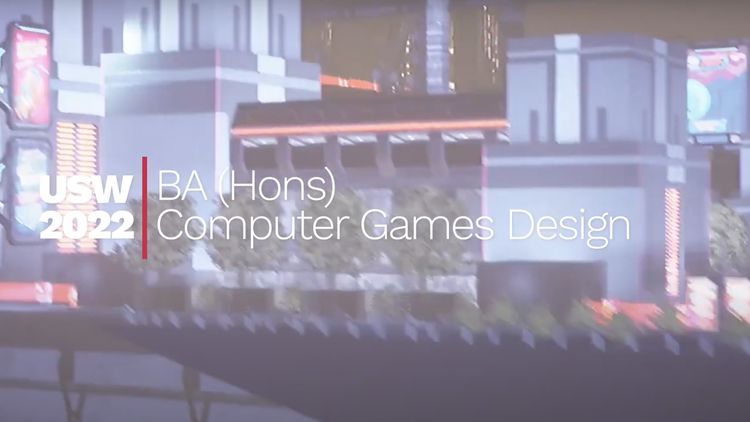The image features a text overlay on a blurry nighttime photograph of a cityscape, possibly an entertainment district. In the background, there are multi-storied, mostly blue buildings with varying shades, some edged in darker blue, and a few adorned with neon signs and advertisements. Some buildings are tall with attached displays, contributing to the urban scene. The text, presented in white characters, is positioned prominently: on the left side, "USW" is written at the top with "2022" directly below it. Separating this text from the rest is a thin, red vertical line. To the right of this line, the text continues with "BA (HONS)" on one line and "Computer Games Design" beneath it. The overall composition suggests a digital or ad-style presentation against the illuminated, high-rise backdrop.